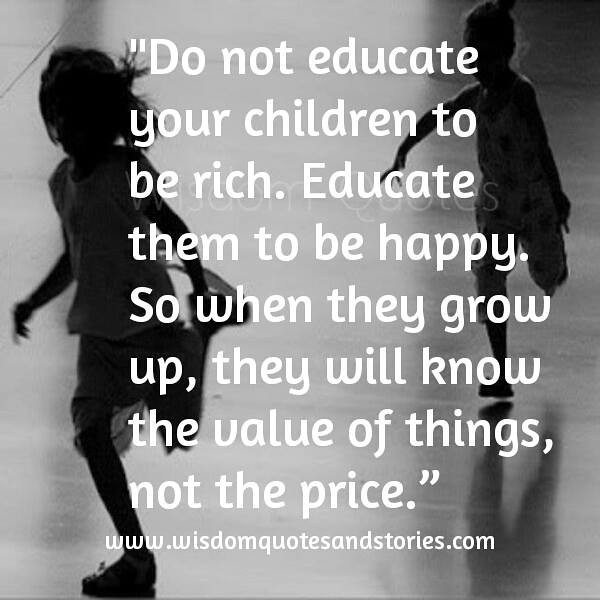The black and white image features a motivational quote prominently displayed in large white letters against a dark, silhouette backdrop. The quote reads, "Do not educate your children to be rich. Educate them to be happy so when they grow up, they will know the value of things, not the price." The backdrop shows the black silhouettes of two children—one running away on the left and the other chasing after on the right. Their features are undefined, making them appear as shadows. Below the quote, the text "www.wisdomquotesandstories.com" is also displayed. The overall scene evokes a sense of timeless pursuit and happiness, framed within a stark yet evocative grayscale palette.